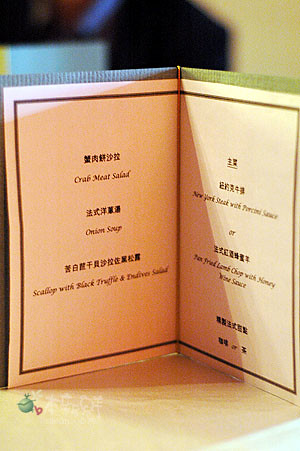In the image, there is an open menu placed against a blurry, out-of-focus background. The menu consists of two white pages bordered with black on the inside. The left edge of the menu is highlighted in blue, while the right edge is accented in green. On the left page of the menu, the first item listed is a crab meat salad, accompanied by text in an Eastern language. Following that is an onion soup listed in the center. At the bottom, there is an entree featuring scallops with black truffle and another solid component. 

The right page of the menu offers a New York Steak with Princess Sauce. Additionally, it lists a dish intriguingly described as "O'er Blank Fox-Fried Lamb Chop with Honey Wine Sauce." At the very bottom left of the page, there is a green circle with white text inside, but the exact wording is not clear. The menu is front-lit, casting a soft gray shadow. The background features a mix of mostly white on the left, black in the middle, and a touch of yellow on the right, adding to the ambiance of the scene.